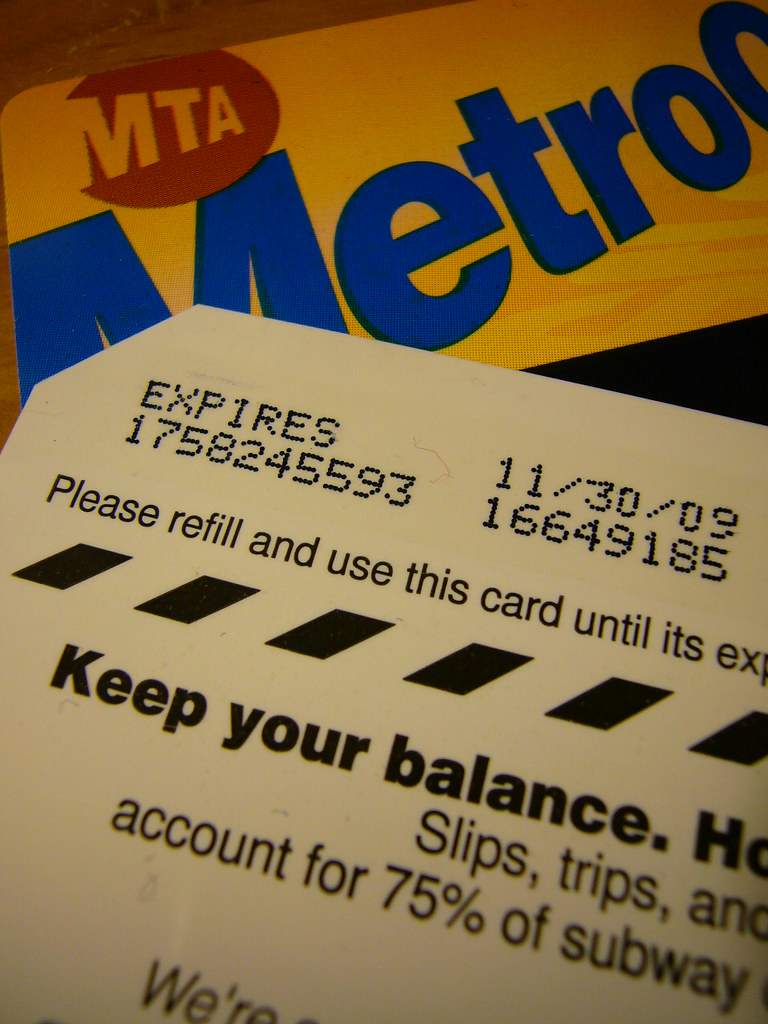The photograph is a close-up shot of two staggered MTA MetroCards. The card at the bottom prominently displays the MTA logo in a red circle and the word "Metro" in blue on a yellow background. Partially covering this card is another MetroCard, which appears to be the back side, featuring a white background with black text. The top portion of this card displays the expiration date "11/30/09" alongside a series of long numerical sequences: "1758245593" and "16649185". Below these numbers, the card instructs, "Please refill and use this card until its expiration date." Further down, partially visible text reads, "Keep your balance. Slips, trips, and falls account for 75% of subway incidents." The photo captures all these elements crisply at the top and middle portions, with some text becoming blurred or cut off towards the edges.